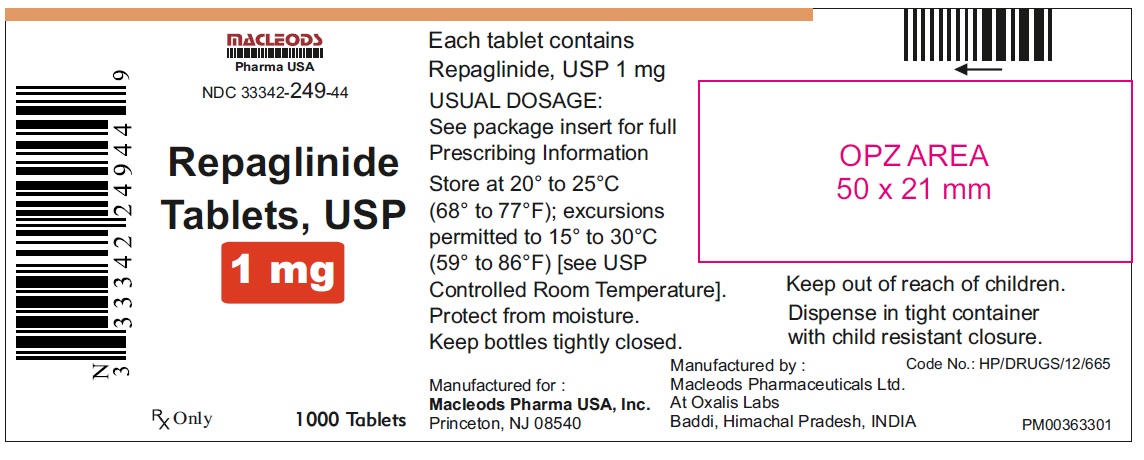This image appears to be a product label for the back of an OPZ area. On the right side, the label features a rectangular black-lined box with a white interior that reads "OPZAREA" and the dimensions "50 x 21 mm." To the left, there is a UPC code prominently displayed. Moving towards the center-right, the label states "REPAGLINIDE" followed by "tablets" and specifies the dosage as "1 milligram." At the top of the label, above these details, the name "McLeod's" is printed, accompanied by a tiny logo resembling "Farmer USA."

The central part of the image seems like a typical layout for a pill bottle label that's been stretched out, showing comprehensive product details. It includes directions for use and a summary of the tablet's contents. An advisory note indicates that the usual dosage can be found by referring to the package insert for full prescribing information.